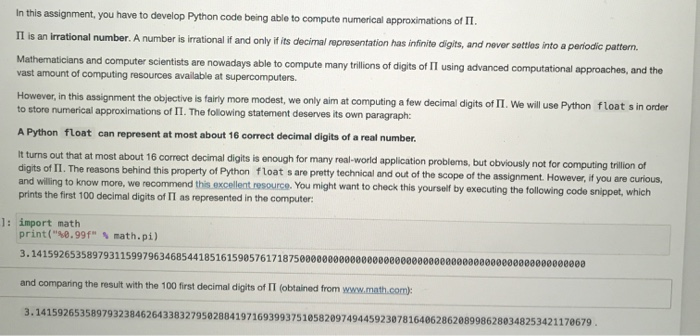**Detailed Caption:**

This is a screenshot containing a significant block of text that outlines an assignment for developing Python code to compute numerical approximations of π (pi). The text explains that π is an irrational number, which means its decimal representation is infinite and does not repeat periodically. While advanced computational methods on supercomputers can now compute many trillions of digits of π, this assignment sets a much more modest goal: computing only a few decimal digits using Python.

The assignment emphasizes using Python floats for storing the numerical approximations of π. A concise yet important statement highlights that a Python float can accurately represent up to about 16 decimal digits of a real number. The assignment notes that while this precision is sufficient for many practical applications, it is inadequate for computing the trillions of digits needed in advanced computations. It also points out that the technical reasons behind this limit are beyond the assignment's scope but encourages students to explore further through an excellent recommended resource.

The image includes a code snippet for students to execute, demonstrating the precision limitations of Python floats. The provided Python code imports the math module and prints π to 99 decimal places. The ensuing comparison reveals fewer decimal places in Python's output versus the first 100 digits of π obtained from an external source like math.com. This comparison reinforces the earlier point about the precision limitations of Python floats.